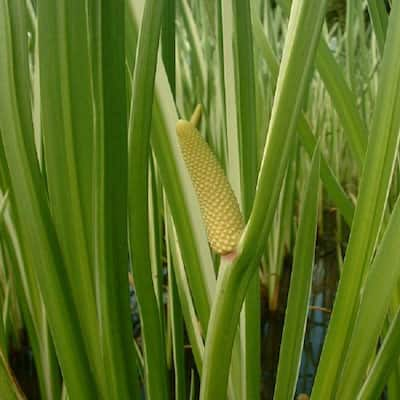The photograph captures a vivid scene of tall, thick, grass-like water plants emerging from a marshy wetland. The plants grow from brownish stems and extend their flat, green blades upward. Dominating the center of the image is a distinctive corncob-like protrusion that is likely the plant's flowering bud. This yellow structure, dotted with gray and slightly bumpy, narrows towards its rounded top. The wetland setting is evident from the visible water at the bottom of the image and its reflective qualities, suggesting the photo was taken outdoors during daylight. The photograph, a perfect square, features a natural palette of green, brown, black, and yellow hues, emphasizing the lush, vibrant environment of the wetland.